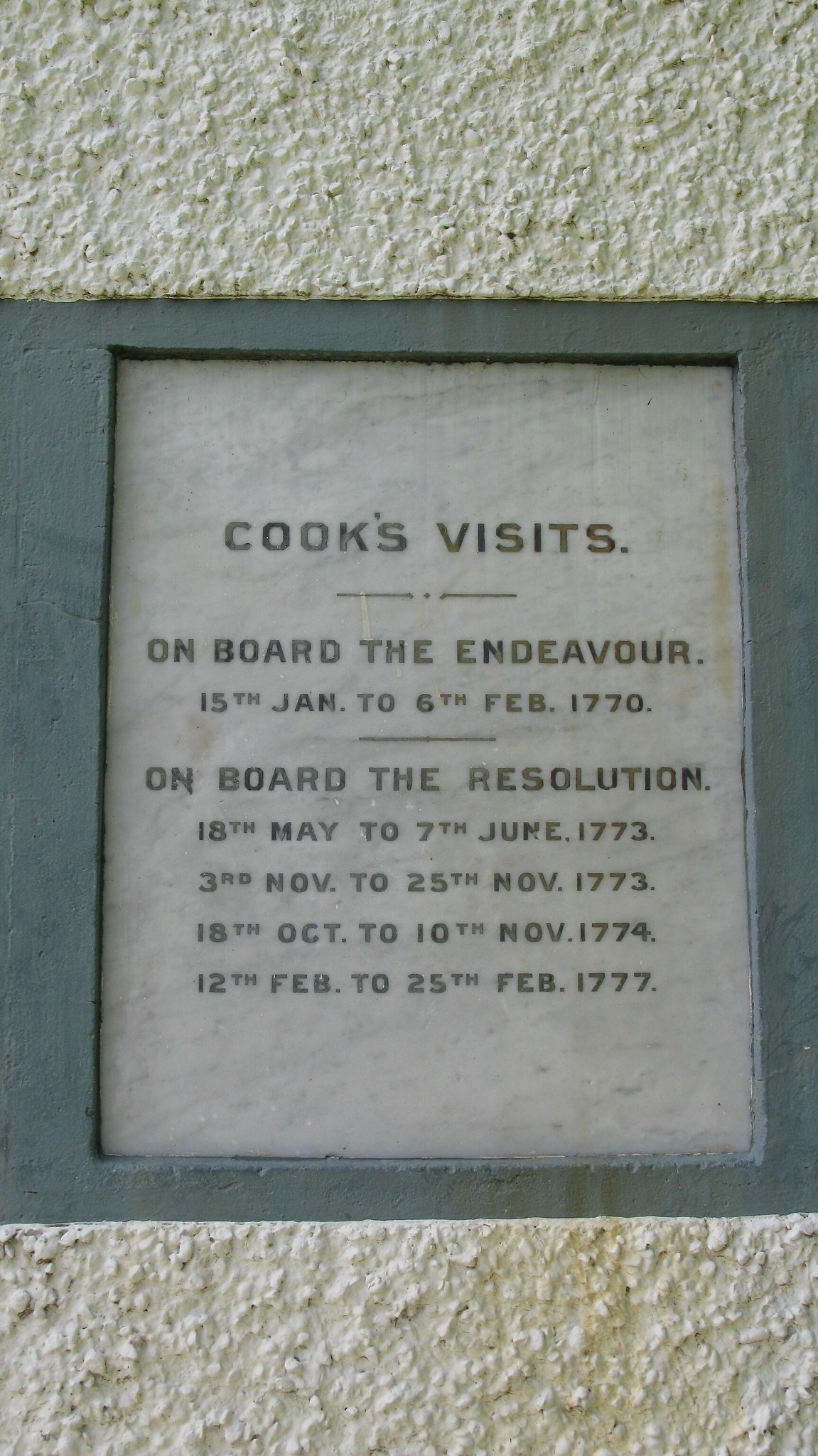This photograph captures a historical outdoor setting featuring a prominently embedded plaque in the side of a building. The plaque, possibly made of marble, is framed by blue, wooden painted pieces, with additional visible elements of a white stucco material and cement or stone wall. The marble plaque is centered in the image and bears the text, "Cook's Visits," detailing the voyages of Captain Cook: "on board the Endeavor, 15th January to 6th February 1770," and several periods on "board the Resolution: 18th May to 7th June 1773, 3rd November to 25th November 1773, 18th October to 10th November 1774, and 12th February to 25th February 1777." The months are abbreviated (JAN, FEB, etc.), and the overall color palette of the photograph includes off-white, green, and tan hues, emphasizing the historical and aged appearance of the setting.